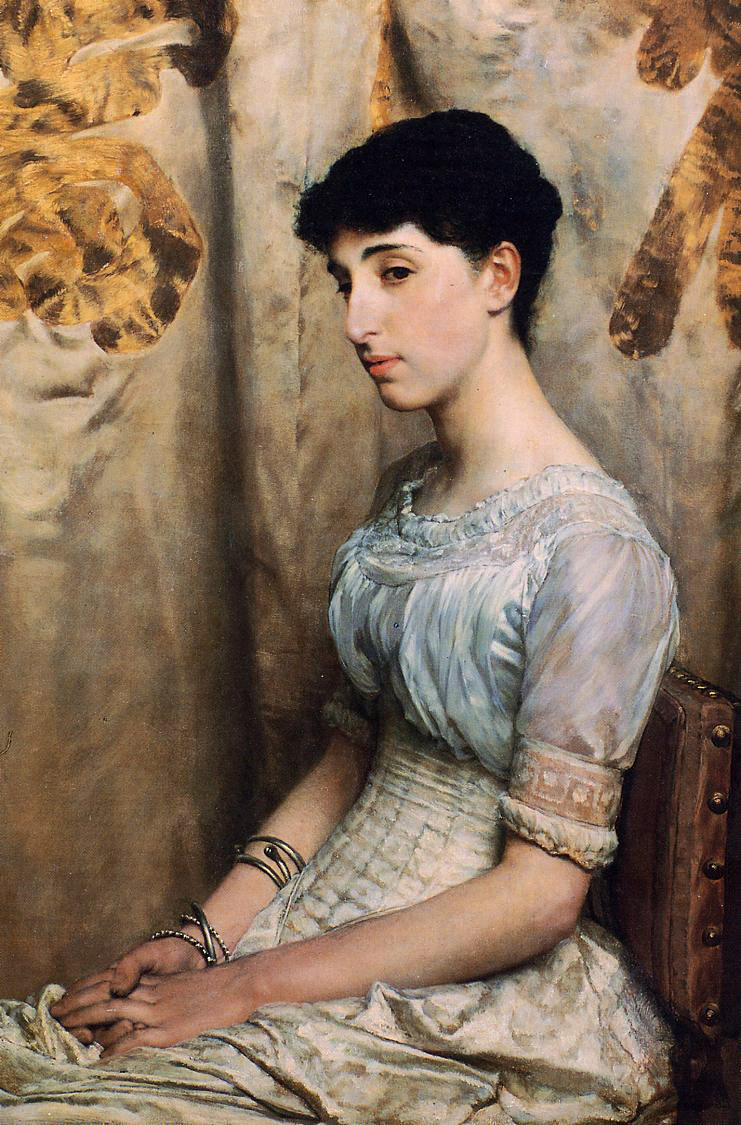The image appears to be a highly detailed painting of a transgender individual or woman, characterized by its realistic and lifelike qualities. The person is seated in a brown leather-backed chair, which features decorative metal studs securing the leather to the frame. Their short, dark curly hair frames a face with a mix of masculine and feminine features, including dark eyes and fair skin.

Dressed in a short-sleeved white dress with a blue corset-like top, the individual has numerous silver metal bracelets adorning their right wrist and forearm. Their hands are gently clasped in their lap, with the right thumb resting over the left hand. The chair and sitter are positioned slightly leftward in the composition, with the person's gaze directed towards the viewer.

The background comprises a warm goldish-brown wallpaper with intricate designs that add to the rich, detailed ambiance of the scene. Additionally, white and gray drapes embellished with a geometric gold thread pattern occupy the upper corners of the image, contributing to the overall depth and complexity of the artwork. The interplay of detailed textures and balanced composition accentuates the lifelike quality of the painting, blurring the lines between painting and photography.